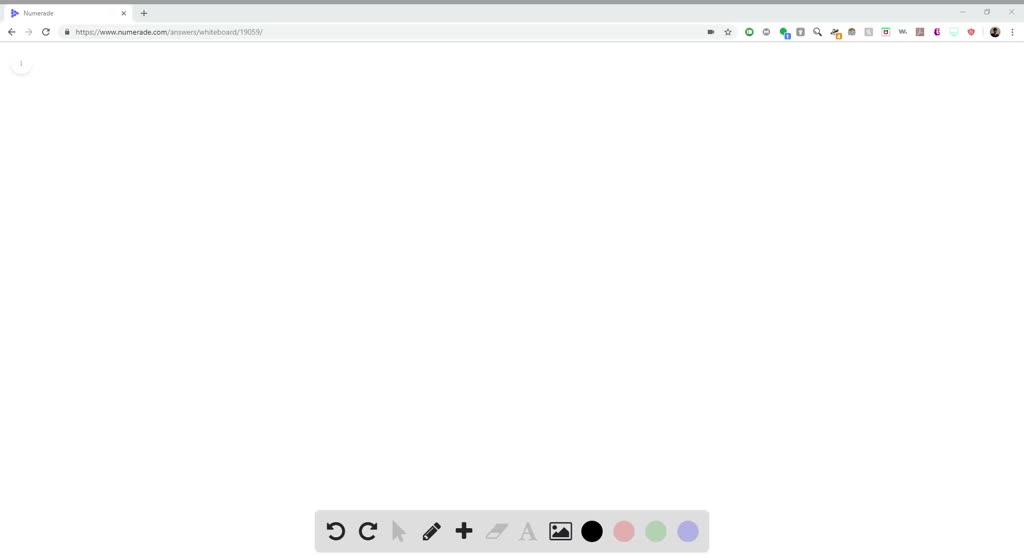The screenshot showcases a website page from Numerade, specifically at the URL "numerade.com/answers/whiteboard/19059/". The interface is viewed through a gray-themed browser, which features a plethora of icons and tools scattered across the page. At the top of the browser tab, various colored circles and squares are visible, including a yellow star, a green circle, a gray circle, another green circle with a Facebook icon, a gray square with a magnifying glass search icon, and an orange square. 

Below the URL bar, another gray toolbar contains navigation icons such as back, refresh, and forward buttons. Additional tools on this bar include a black cursor tool, an edit plus icon, a font tool designated by the letter 'A', a photo upload icon, and a set of colorful circles in black, pink, green, and purple - likely for color options. 

The main body of the website, however, remains blank, signified by a vast white field with no visible content. This emptiness suggests that the page content failed to load or is otherwise not displayed. The user has no prior experience with this site, leaving them unable to discern the website's purpose or functionality from this view alone.